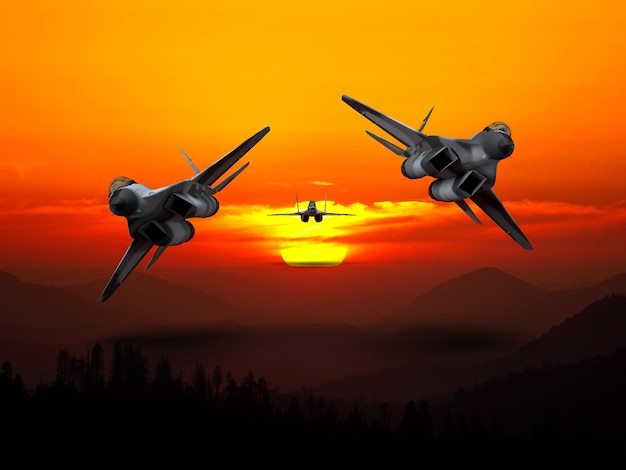The digitally created image depicts a dramatic aerial scene featuring three fighter jets. Against the backdrop of a vibrant sunset, the sky is painted in deep hues of orange, red, and yellow, gradually fading into lighter shades toward the top. The jets, camouflaged in shades of white, gray, and green, dominate the upper section of the image. Two jets are in the foreground, banking sharply in opposite directions — one towards the left and the other to the right — suggesting dynamic movement. The third jet follows a straight path, aligned centrally above the incandescent setting sun, which partially obscures the darkened forest and rolling hills below. The landscape, though silhouetted and shadowed, reveals layers of mountains and tree tops, adding depth to the serene yet intense atmosphere of this digital artwork.